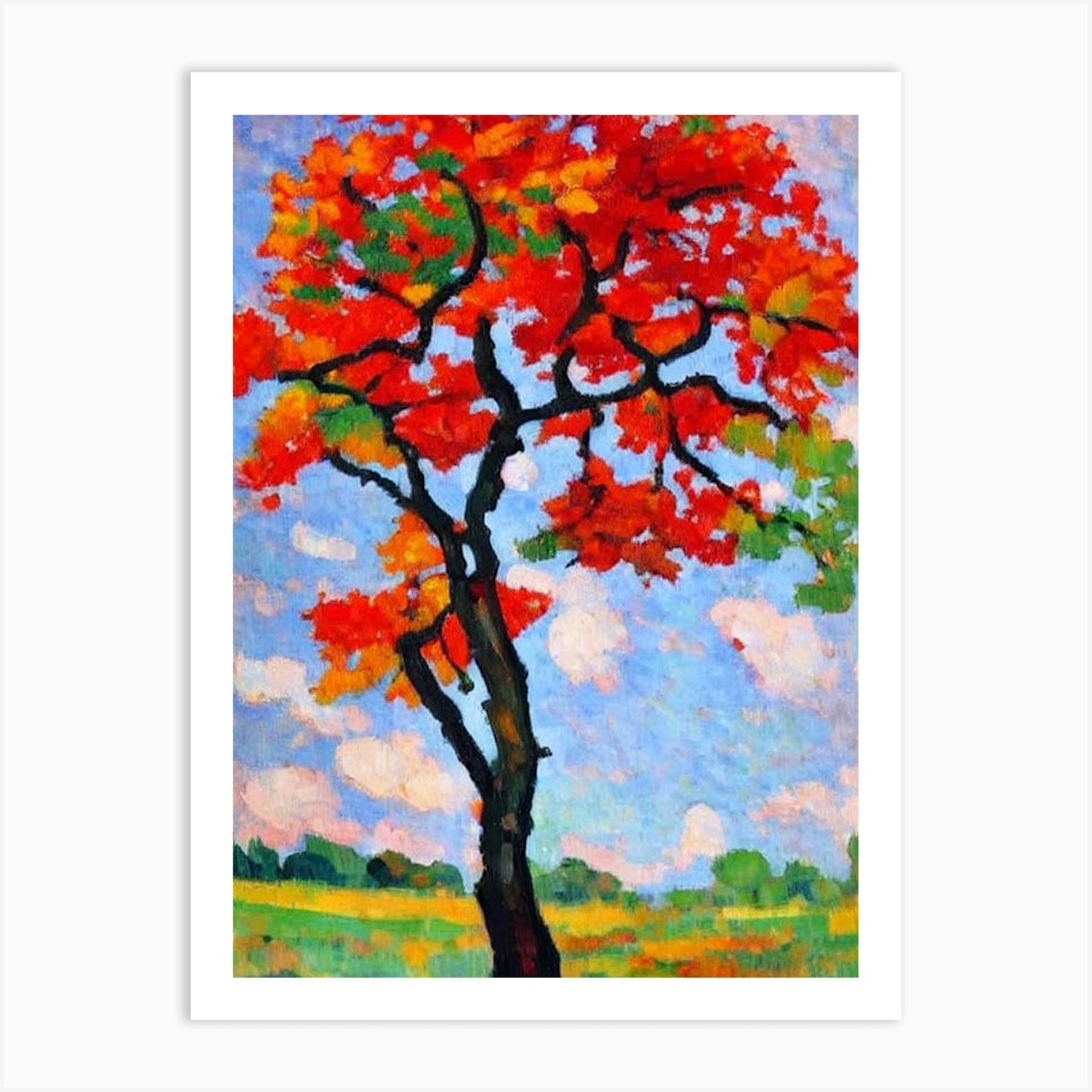The image is of a vibrant autumn scene captured in a painting, bordered by a white frame and presented as a vertical art print with a slight drop shadow. The artwork appears to be done in acrylic or oil, characterized by thick, padded strokes. 

At the center stands a dark brown to black tree trunk with grayish-teal and brown highlights, extending from the bottom to the upper parts of the painting. The branches are adorned predominantly with deep red leaves, reminiscent of candy apple red, interspersed with shades of orange, green, and yellow, creating a vivid canopy that spans the upper portion of the image. 

Below the tree, the ground is a green and yellow field suggestive of the fall season, stretching toward the horizon where there are splotches of green bushes and smaller trees. Above this landscape stretches a light blue sky filled with white fluffy clouds, some tinged with pinkish and peachish hues, completing the serene backdrop.